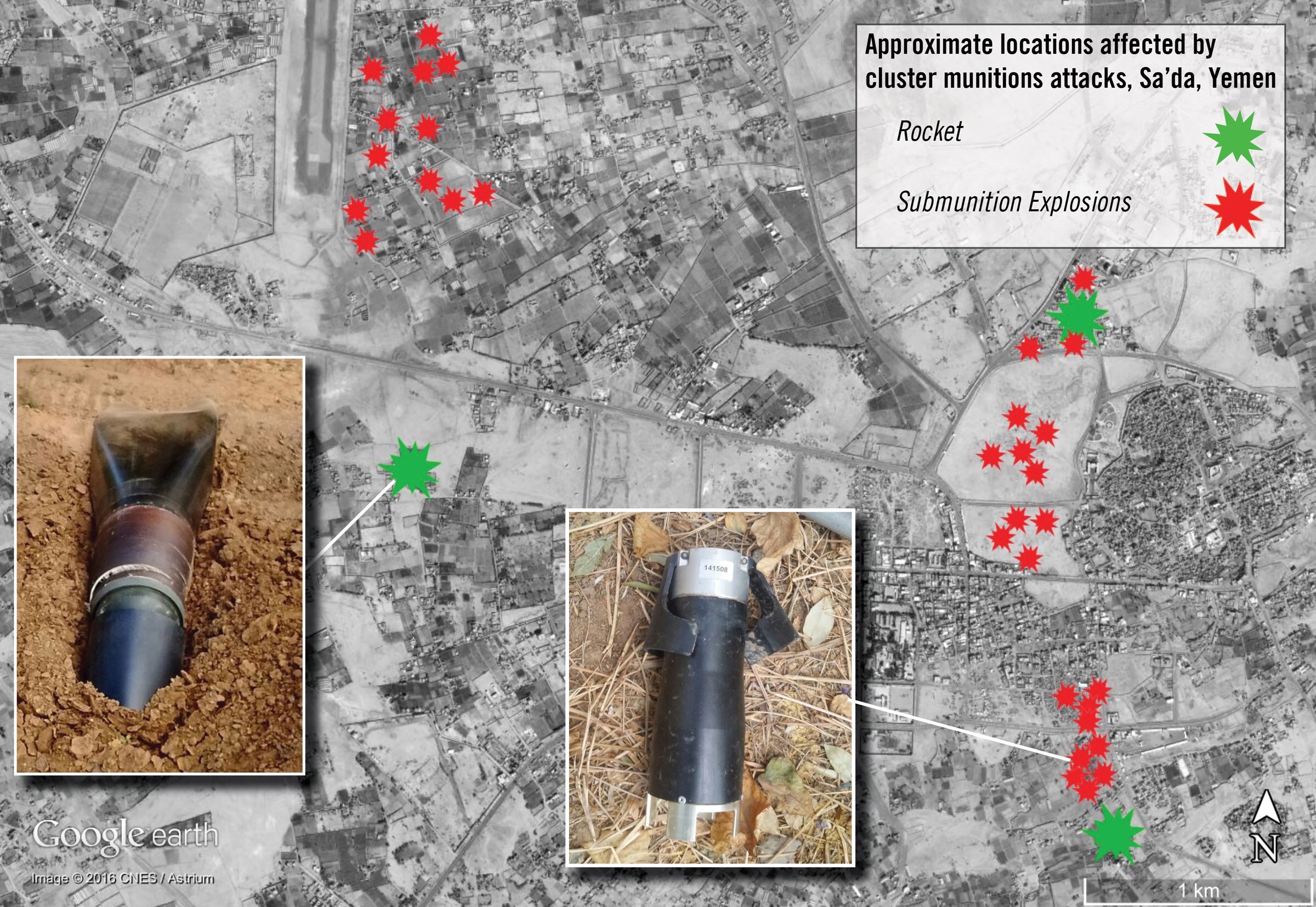This image is an overhead, black and white map of Saada, Yemen, sourced from Google Earth (2016 CNES). It is titled "Approximate Locations Affected by Cluster Munition Attacks" in the upper right corner, and includes a key that explains the symbols: green stars indicate rocket attacks, while red stars signify submunition explosions. The map is speckled with numerous red stars predominantly on the right-hand side, with a few green stars scattered around. 

Inset into the map are two close-up photographs. The left inset shows a rocket, partially buried in the dirt with a shape reminiscent of a vacuum cleaner attachment, having a black and brown color. The right inset displays a submunition, resembling a flashlight with a black body and silver top, lying on some hay. These provide real-world imagery of the munitions depicted symbolically on the map.

The overall context indicates a residential area, marked by numerous dots corresponding to affected locations, highlighting the impact of the conflict in this region of Yemen.